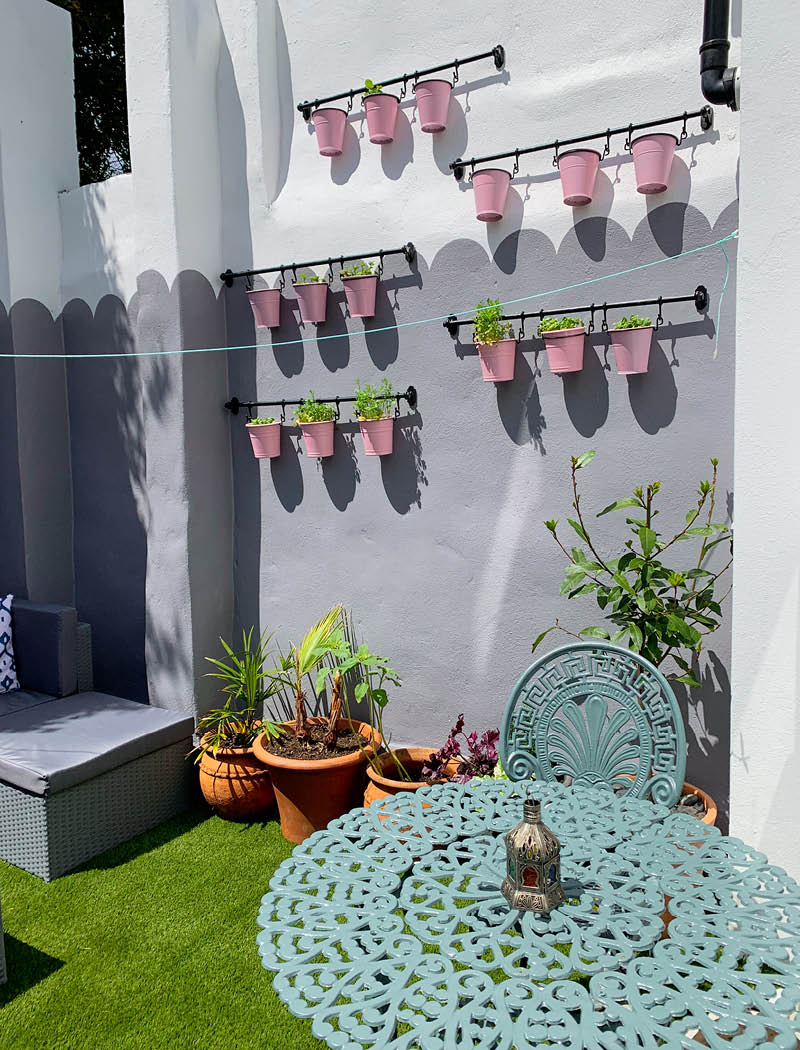This photograph showcases the exterior of a building with a stucco texture. The wall is divided horizontally into two parts: the bottom section is gray and adorned with a series of semicircular patterns, and the upper portion is white, except for a lavender section beneath the white, separated by scalloped edges. Rectangular vertical pillars extend from the wall, suggesting possible doorways without visible doors.

Attached to the wall are five black horizontal metal bars, staggered and each holding three pink flower pots suspended by chains. Some of these pots contain green foliage, while others are empty. At the base of the wall, there are large clay pots with various plants growing in them.

In front of this setup, there's a teal-colored, intricately patterned wrought iron bistro table accompanied by a matching chair. A silver centerpiece adorns the table's surface. Additionally, a wicker bench painted the same color as the wall is situated nearby, along with gray outdoor upholstery. The ground is covered with closely manicured, vivid green grass. The scene is illuminated by bright sunlight, indicating it is daytime, and the overall ambiance suggests a serene, well-maintained garden or lawn area.